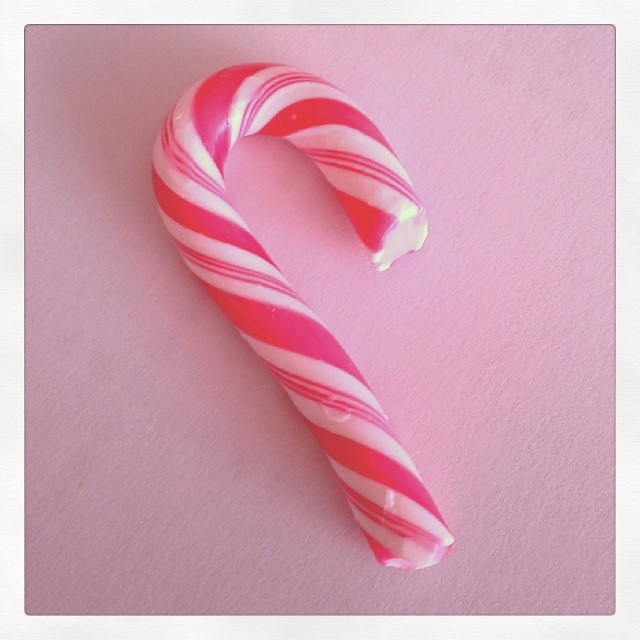This square-shaped image, bordered with a half-inch white frame, showcases a close-up view of a small candy cane resting diagonally on a flat, bubblegum pink background that appears slightly brighter on the right due to shadowing. The candy cane itself is predominantly pink with white stripes and features noticeable wear: the curved top section and the straight bottom portion both exhibit bite marks and notches. Melted and ridged areas are evident where someone has sucked on and snapped pieces of the candy cane. The pinkish hue of the candy contrasts against the lighter pink backdrop, with some glare visible near the top, enhancing the intricate details of the candy cane's texture.